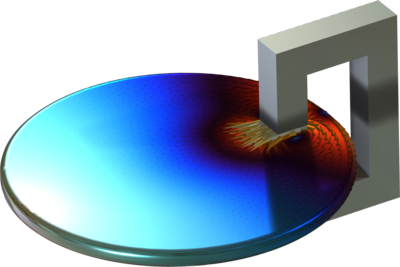In this image on a white background, there is a 3D-rendered scene featuring a disc and a unique gray structure. The disc is situated towards the upper left and displays a gradient of colors, transitioning from aquamarine on the left, through blue in the middle, to red on the right edge. This colorful disc is being held or clamped by a vertical, C-shaped gray block located on the right. The block, which resembles an incomplete rectangle with a hollow rectangular center, appears as though it is made of concrete. Scattered along the blue area of the disc are some small, gray dots. Shadows and shading are present, adding to the 3D illusion of the image. This scene looks like an abstract stock image, likely intended to represent some form of modern art or design.